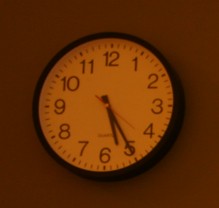This photograph captures a small, square-shaped image of a clock, measuring approximately three inches on each side. The clock is mounted against a dark burgundy, almost black, background, contributing to the overall dim and moody atmosphere of the scene. The lighting is poor, likely due to a lack of natural light or nighttime conditions, casting deep shadows over the clock. 

The clock itself is circular with a pronounced black outline. Its face features bold black numbers ranging from 1 to 12. The timepiece includes three distinct hands: the hour and minute hands are black and relatively thick, while the second hand is red and exceptionally thin. The clock displays the time as approximately 6:25.